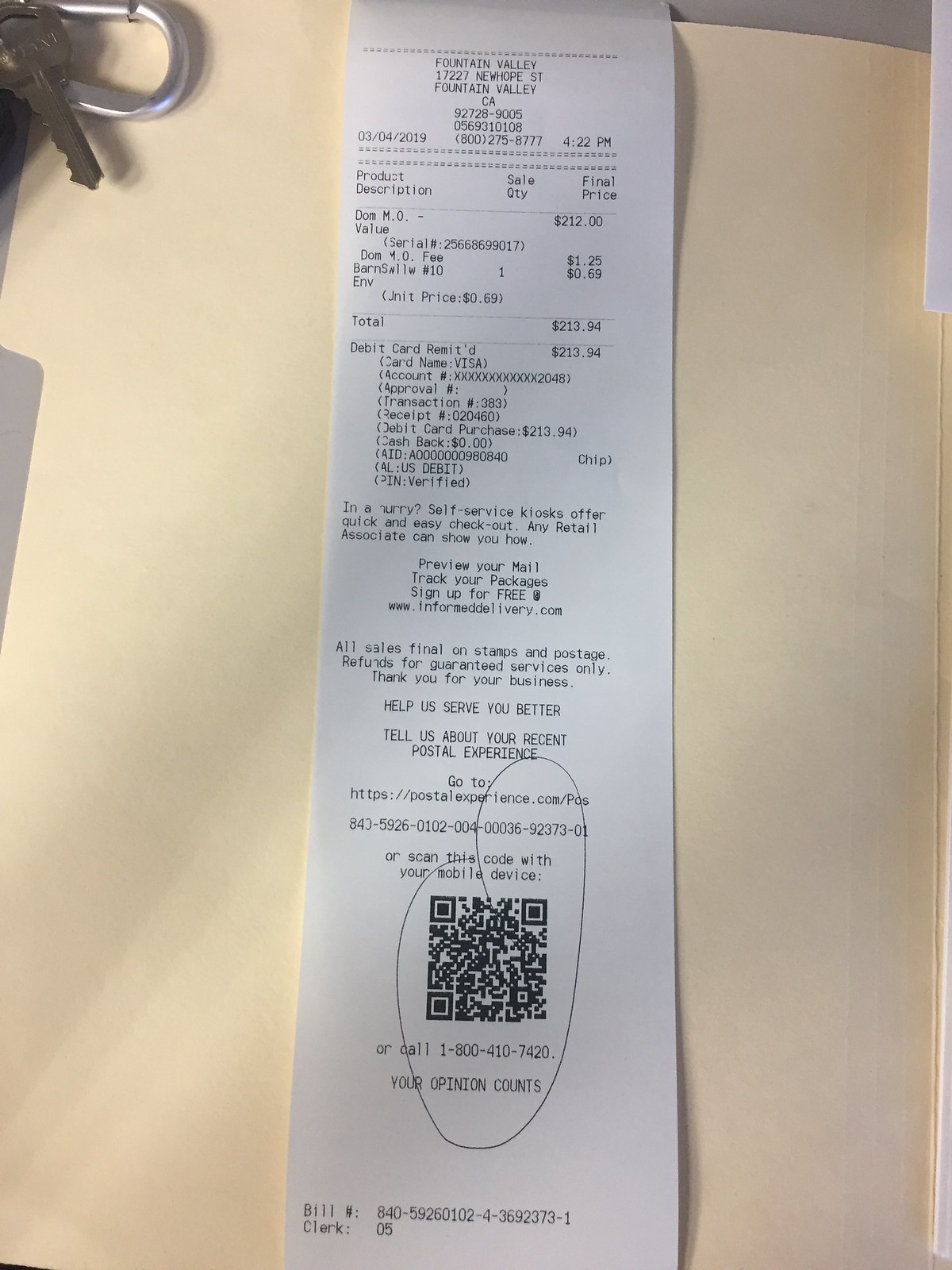A close-up photograph capturing a detailed view of a receipt issued on white paper with black font. The receipt lays flat on a pristine white table. In the upper left corner of the image, a silver keychain with a bronze key is partially visible, casting a distinct shadow onto the table surface.

The receipt prominently displays the business name and address at the top, followed by the date and time of the transaction. The sale price, alongside debit card details including the cardholder's last name and the card number, is clearly printed. A note advises customers that self-service kiosks are available for those in a hurry. The receipt also emphasizes that all sales are final and includes a feedback request, encouraging customers to share their recent postal experience to help improve service.

Near the bottom of the receipt, a black QR code is circled for emphasis. Directly beneath the QR code, a phone number is provided for further assistance or inquiries.